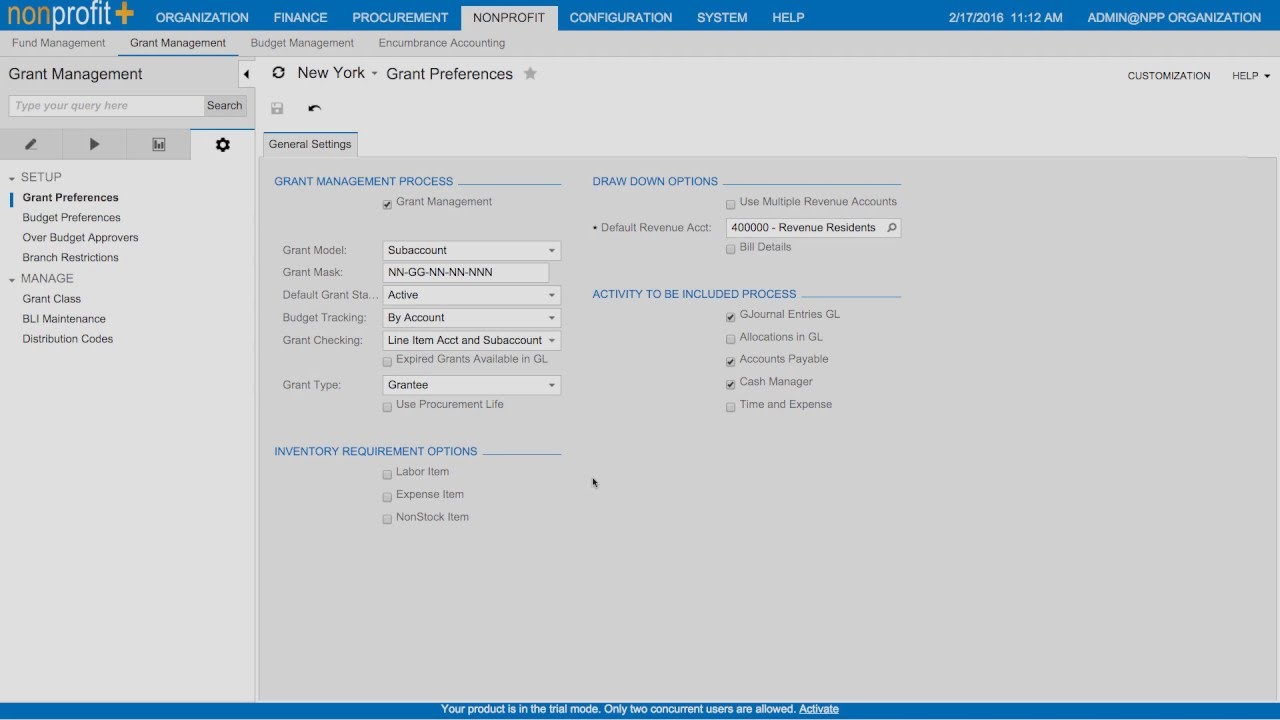**Caption:**

The image showcases a detailed view of a non-profit organization's web page, dated December 17, 2016, at 11:12 AM. The interface includes several pivotal tabs at the top, such as Organization, Finance, Procurement, Non-Profit (the current active section), Configuration System, and Help. On the far right, there's an admin panel marked as "Admin at NPP Organization."

Directly below, the user is focused on a particular section under 'Grant Management,' which is indicated by the active left sidebar tab. This section also contains other related tabs like Fund Management, Budget Management, and Encumbrance Accounting. 

Within the 'Grant Management' area, there is a search box, followed by setup options such as Grant Preferences, Budget Preferences, Local Budget Approvers, Branch Restrictions, and a Manage section. This section lists items like Grant Class, BLI Maintenance, and Distribution Codes.

To the right, under the heading "New York Grant Preferences," there is a General Settings tab that further expands into four distinct sections:
1. **Grant Management Process:** This includes elements like Grant Model, Grant Mask, Default Grant, Budget Tracking, Grant Checking, and Grant Type.
2. **Inventory Requirement Options:** Options here consist of Labor Item, Expense Item, Non-Stock Item, all featuring checkboxes.
3. **Drawdown Option:** It displays the Default Revenue Account, which contains an entry of 4 million revenue residents.
4. **Activity to Be Included Process:** This section has several checkboxes with the following options: G Journal Entries (checked), GL Allocations in GL (unchecked), Accounts Payable (checked), Cash Manager (checked), and Time and Expense (unchecked).

The entire layout provides a comprehensive management interface for handling various aspects of grant administration for the non-profit organization.